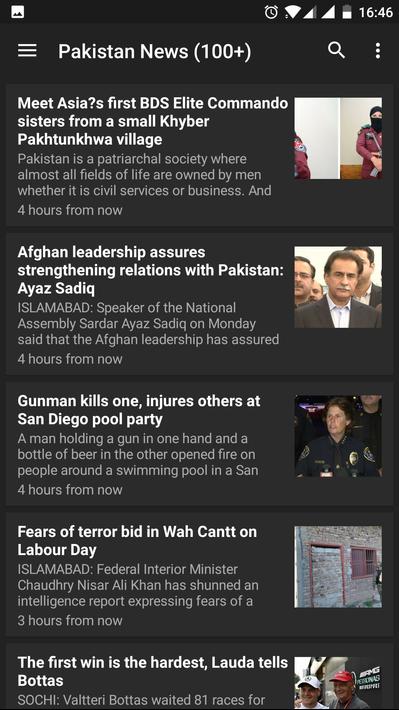On this smartphone screenshot, captured with a black background, there's a series of status icons displayed at the top. On the upper right, a white alarm icon, Wi-Fi icon, dual network icon, battery icon, and the current time, 16:46, are visible. To the upper left, a colored screenshot notification icon stands out amidst the white icons. Centered below these icons, the text reads "Pakistan News 1000+," with a search icon to its right and a menu icon (three horizontal white lines) to its left.

Beneath the "Pakistan News" heading, several news articles are listed, each accompanied by an image on their right. The first article headline reads, "Meet Asia's First BTS Elite Commando Sister from a Small Kiba Pakchunkwa Village," highlighting the rarity of women in such roles within Pakistan’s patriarchal society. This article was posted four hours ago. 

The second headline states, "Afghan Leadership Assures Strengthening Relations with Pakistan: Ayaz Sadiq," reflecting ongoing diplomatic engagements. The timestamp indicates it was also posted four hours ago.

The third headline covers a tragic event: "Gunman Kills One, Injures Another at San Diego Pool Party," also noted as being posted four hours ago.

The fourth article discusses security concerns: "Fear of Terror Paid in War Count on Labor Day," published three hours ago.

Finally, the fifth article reads, "The First Win is the Hardest: Louder Tales Bought Us," detailing challenges overcome, accompanied by relevant images.